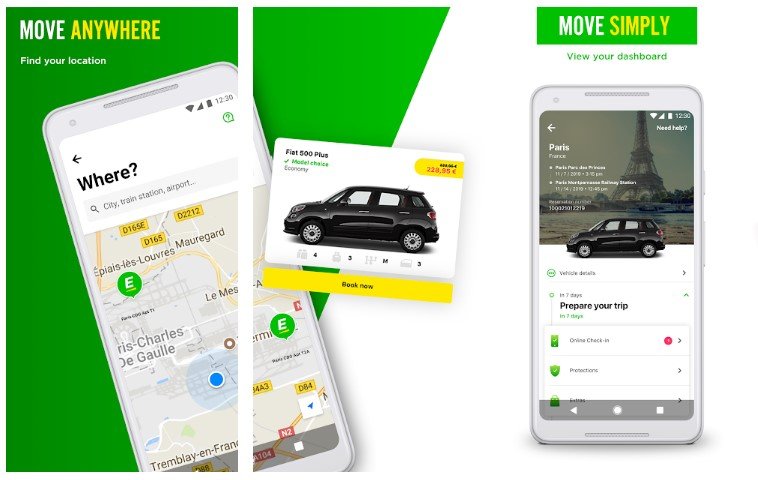**Detailed Caption:**

This digital advertisement, likely for a moving company or travel service, is shown as a computer screenshot. Dominantly featured in the upper left corner are the words "Move Anywhere" followed by "Find Your Location." A light gray smartphone is tilted slightly and positioned towards the left side of the image, angled diagonally towards the right. The phone's screen displays the text "Where" situated in a white box at the top, with a map of Paris underneath, identifiable by landmarks such as Charles de Gaulle Airport.

Adjacent to the phone, to its right, is a small white box overlapping slightly onto the phone's display. Inside this box is an image of a black Fiat 500 car oriented to the left. Above the car, the text "Fiat 500 + Model Choice Economy" is prominent, and to the upper right within the box, there is a yellow rectangle displaying a price. Below the image of the car, a prominent yellow bar spans the bottom of the white box with the words "Book Now."

To the far right of the advertisement, another light gray smartphone is displayed at the top right corner. The screen of this phone shows an image labeled "Paris," featuring the Eiffel Tower with the black Fiat 500 situated in front of it. Beneath this image, additional options are noted, including "Prepare Your Trip" and "Online Check-In," suggesting interactive elements to assist with travel preparation.

The advertisement employs a color scheme transitioning from green to white; the left half of the image has a green background, while the right half features a mostly white background. In the top right corner, the text "Move Simply" is followed by "View Your Dashboard," reinforcing the ease of use and accessibility of their services.